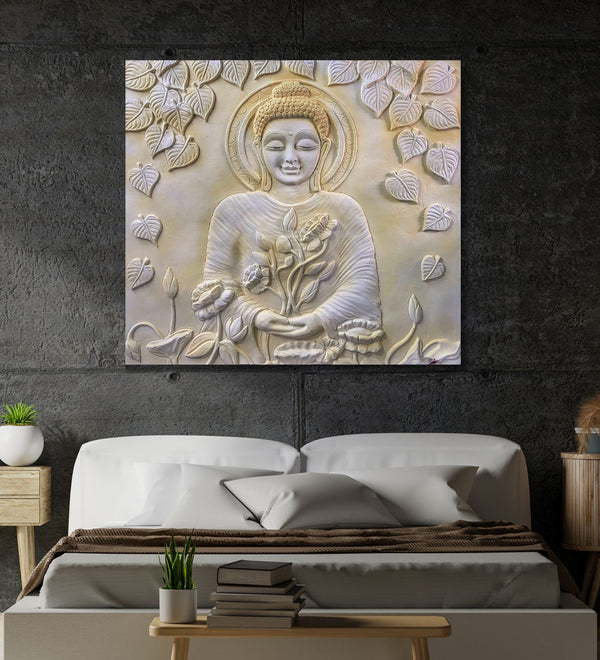This photograph captures the interior of a serene bedroom featuring a centrally placed platform bed adorned with white pillows and a brown blanket. Flanking the bed are two wooden nightstands, each with a vibrant green plant. At the foot of the bed, a small wooden end table holds a stack of books and a succulent in a white planter. Dominating the gray, concrete-like stone wall above the bed is a large wall hanging—an intricately detailed metal or stone relief of Buddha, painted in shades of white, yellow, and tan. Buddha holds plants in his hands, surrounded by flowing leaves and a subtle halo behind his head, giving the artwork an old-time, religious aura.